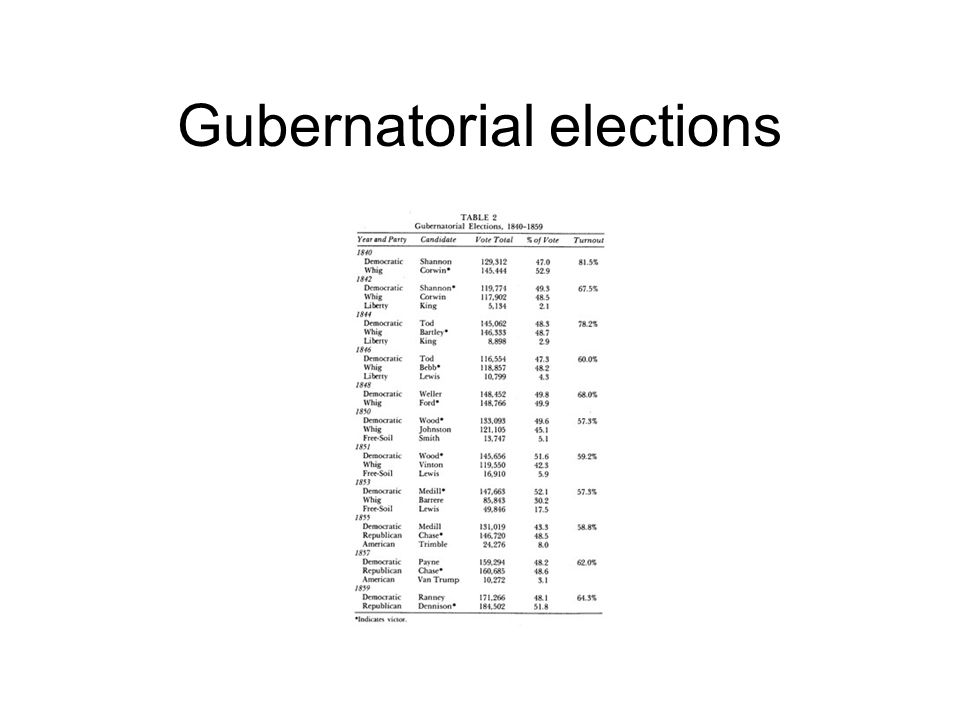The image features a detailed, borderless chart on a white background, prominently titled "Gubernatorial Elections" in large black print. Below the title, a smaller header reads, "Table 2, Gubernatorial Elections, 1840-1859." The table beneath is organized into five columns: Year and Party, Candidate, Vote Total, Percent of Vote, and Turnout. Each column systematically lists yearly data from 1840 to 1859, with separate categories for political parties such as the Whigs, Democrats, Liberty, Free Soil, Republican, and American. The data comprehensively covers each party's candidates, their vote totals, voting percentages, and voter turnout for each election year within the specified period.